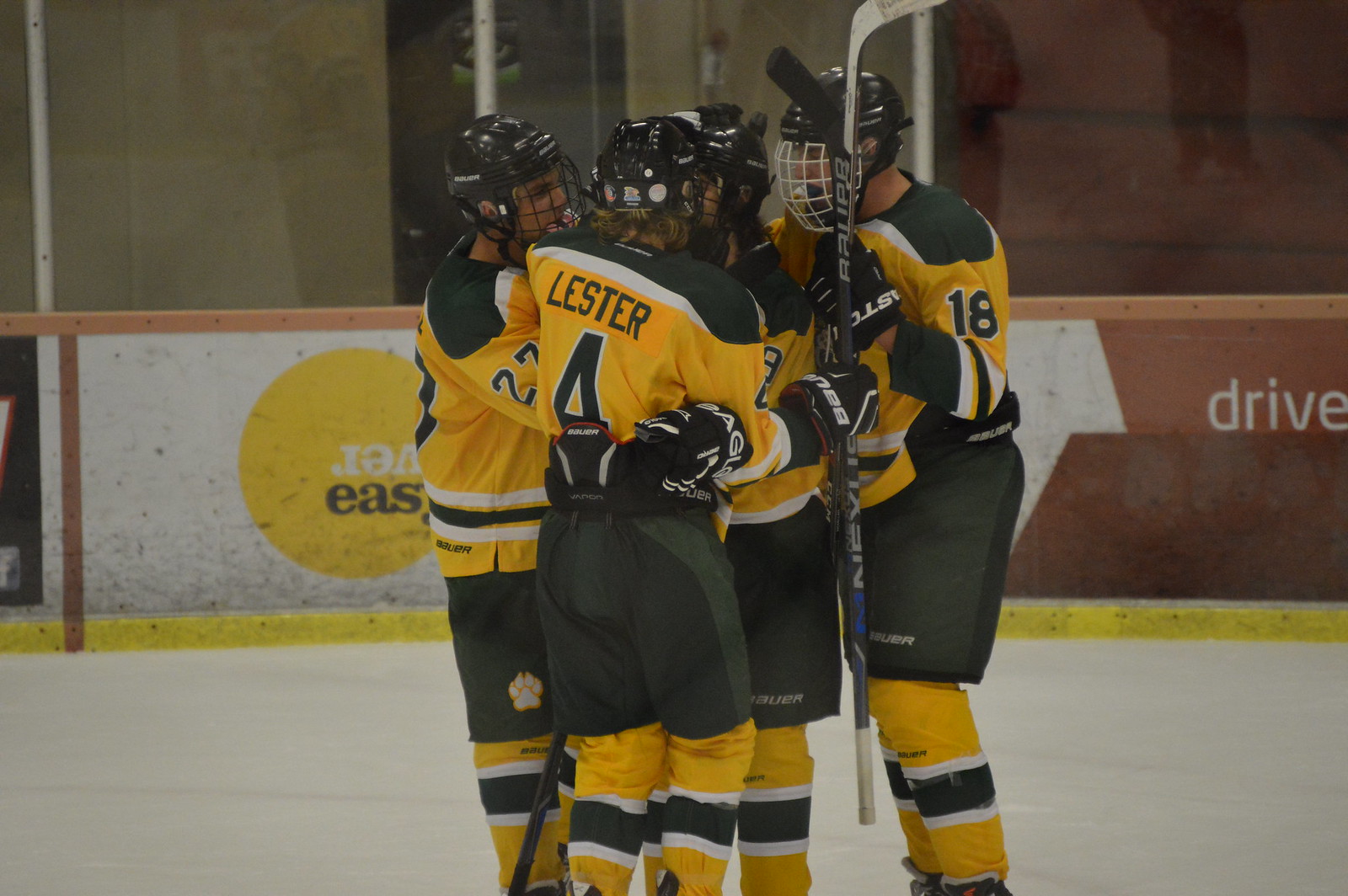The image depicts a rectangular photograph taken during or after a hockey game, centered on a group of hockey players. The scene shows at least four to six players huddled together in an intimate, celebratory embrace. Dressed uniformly in black and yellow gear, the players appear to be part of the same team, sporting black helmets and adorned with distinct paw print designs on their shorts, suggesting a bear motif. One player, distinguishable by a face guard, likely serves as the goalie. They all hold their hockey sticks as they gather on the ice, perhaps discussing strategy or celebrating a victory. The background reveals a brown and yellow wall with a white stripe at the bottom, and partially visible, unreadable words. Above the boards with the usual sponsors and advertisements, there's plexiglass, and beyond, a wall with a door and the start of what seems to be the stands, though no fans are visible in the shot.